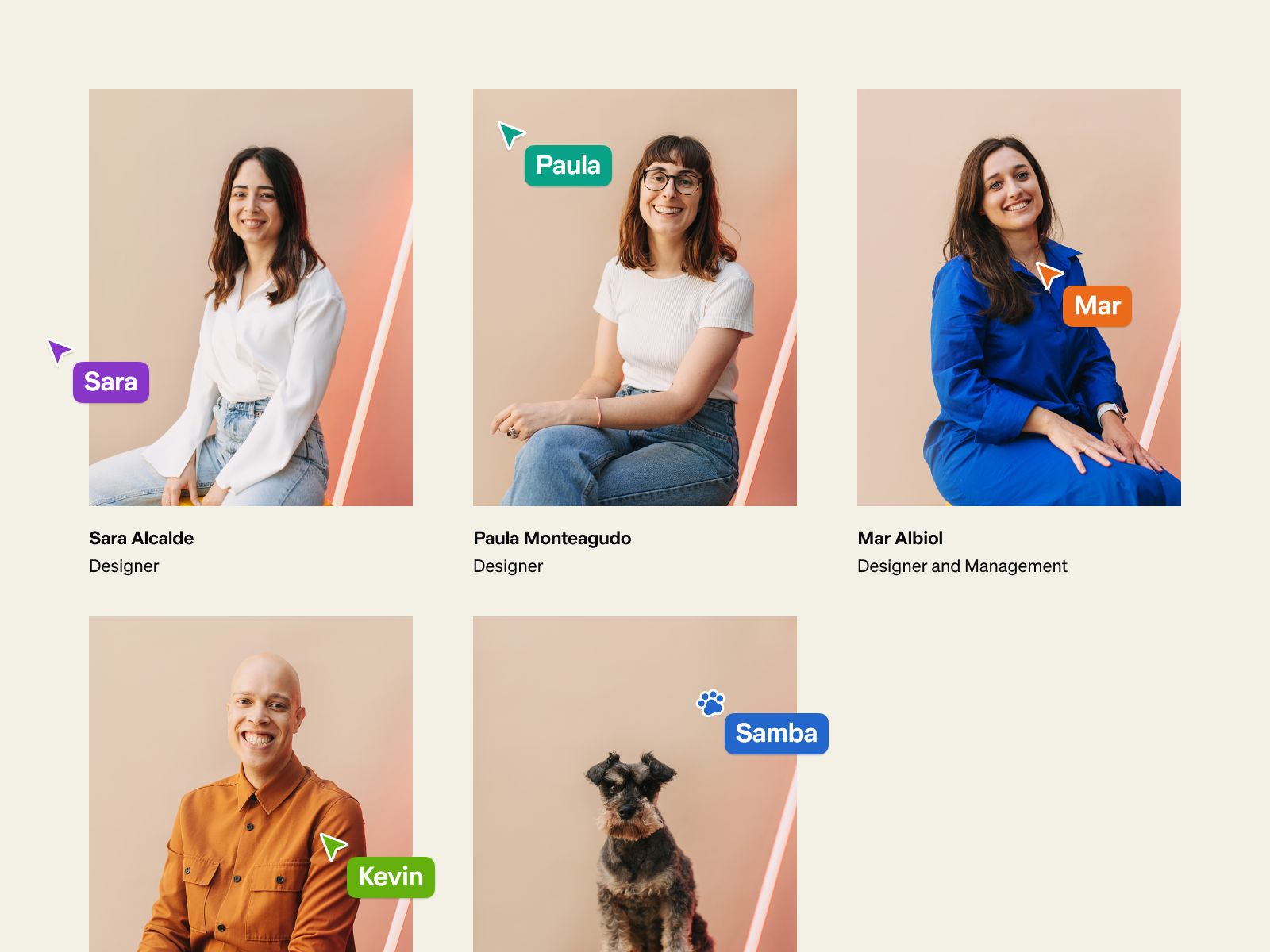The image features a collage of five distinct photos, three on the top row and two on the bottom row, set against a gradient backdrop that transitions from light peach in the upper left corner to a darker peach in the lower right. A diagonal line separates the photos, running from the center-right to the bottom.

In the top row:

1. **Sarah Alcalde**: She is a designer dressed in a white, long-sleeve shirt and blue jeans. Sarah has dark brown hair that falls to her shoulders and stands out against the background with her serene and focused expression.
   
2. **Paula Monteagudo**: Also a designer, Paula is seen in a white short-sleeve shirt. She sports shoulder-length hair and glasses, portraying a balanced and intellectual demeanor.

3. **Mara Albiól**: Wearing a blue top, Mara is described as a designer and manager. Her long hair cascades past her shoulders, adding a touch of elegance to her professional appearance.

On the bottom row:

4. **Kevin**: The image of Kevin is slightly cropped, revealing his bright, engaging smile. He is bald and wearing an orange shirt, exuding a cheerful and approachable aura.

5. **Samba**: Adjacent to Kevin is Samba, a schnauzer dog. Though the photo is also partially cropped, Samba's distinctive features, such as its expressive eyes and prominent beard, are clearly visible.

The collage seems tailored for a professional website, providing a snapshot of the team members and their roles within the organization.